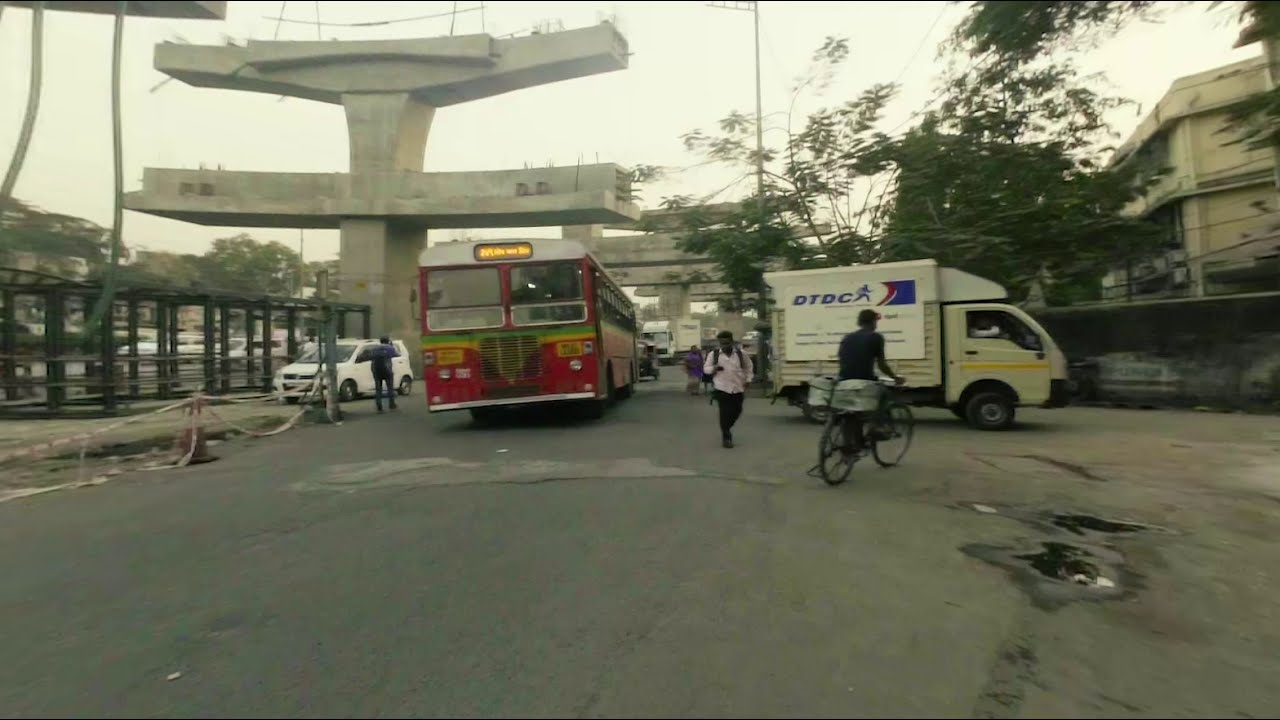This is a detailed photograph of a bustling city street. Prominently in the center of the image, a large red bus with green and yellow stripes is heading towards the viewer, its front portion clearly visible with destination signs blurred but lit in yellow. To the left of the bus, a man with a black backpack appears to be talking on his phone. Behind him, a white minivan is spotted. On the right side of the bus, there is a man in a light pink shirt, black pants, and backpacks walking towards the camera, with a cyclist nearby riding a bicycle that has two squarish pouches. Further in the background on the right, a company van branded "DTDC" is visible, moving to the right side of the frame.

The road is populated with diverse types of vehicles, including a mini-truck carrying the DTTC logo. Pedestrians are seen walking along the street, adding to the liveliness of the scene. On the left side of the road, there are semi-constructed freeway pillars indicative of ongoing construction work, with buildings and trees lining this side as well. The right side features more trees, buildings, and a wall, creating an urban landscape. The sky above appears white, completing the backdrop of this everyday city scene.